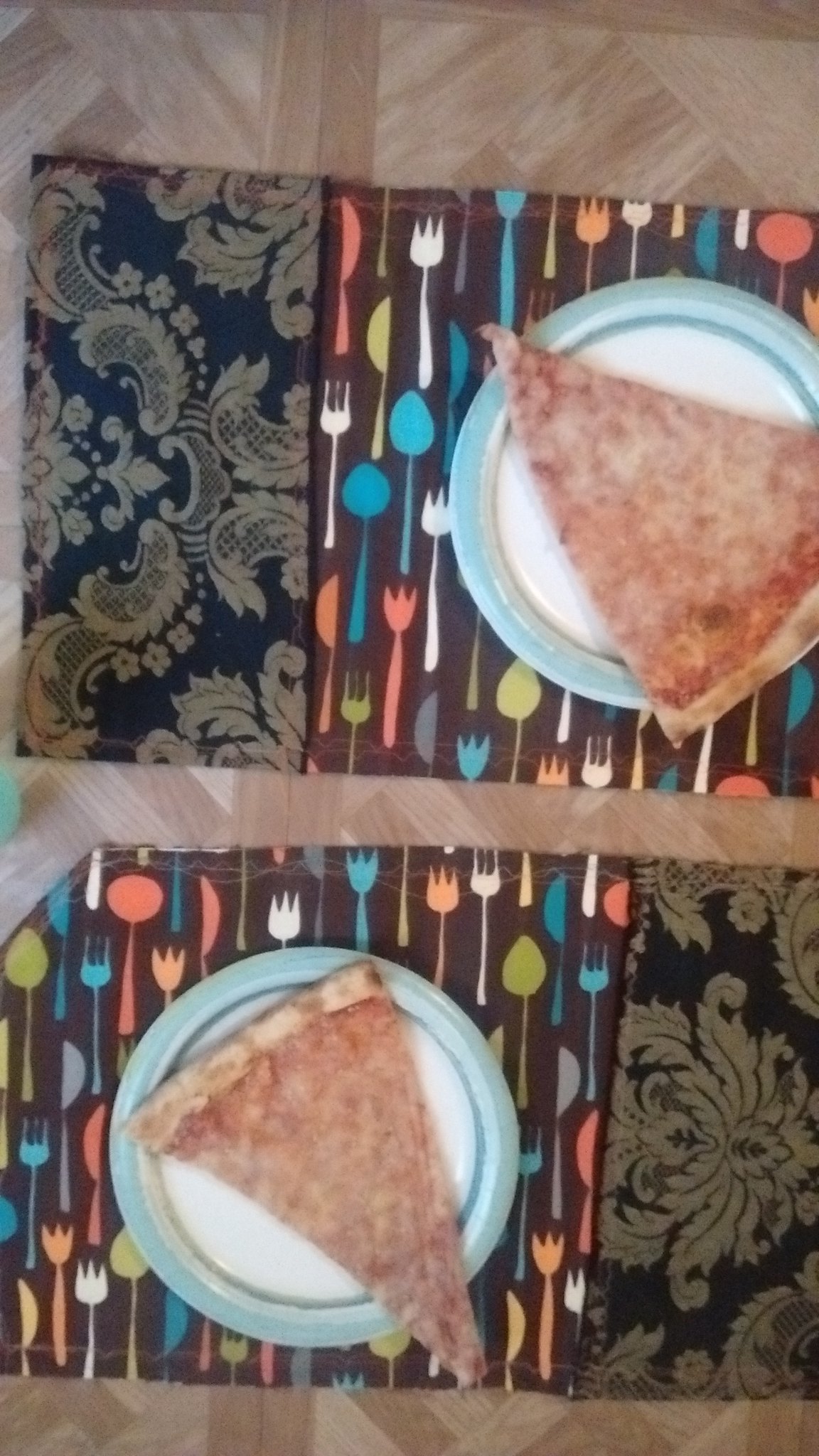The image is an overhead color photograph, slightly out of focus and low in quality, taken in a portrait orientation, likely with a smartphone. It captures two place settings on a brown wooden table. Each setting features a vibrant, rectangular placemat with a dark background adorned with multicolored cutlery—white forks, blue spoons, green knives, orange knives, and pink forks. Additionally, there is a decorative black border on one side adorned with a gold floral fleur-de-lis design.

On top of these placemats are disposable-looking plastic plates, each with a white center, a light blue outer rim, and a darker blue inner ring. Each plate holds a single slice of cheese and tomato pizza. The pizza slices are large and extend off the plates: the bottom slice is oriented with its tip pointing towards the 4 o'clock position and hanging off the plate's edge, while the top slice points upwards towards the 10 o'clock position, with its bottom crust directed towards the 8 o'clock position. Notably, the plate in the top right is partially cut off by the frame of the image. 

Both place settings are positioned vertically, one above the other, with the top plate set slightly towards the right and the bottom plate slightly towards the left. The contrast of the multicolored cutlery against the dark placemats, along with the distinct blue-rimmed plates and the appetizing slices of pizza, creates a visually detailed and engaging composition despite the image's lower quality.